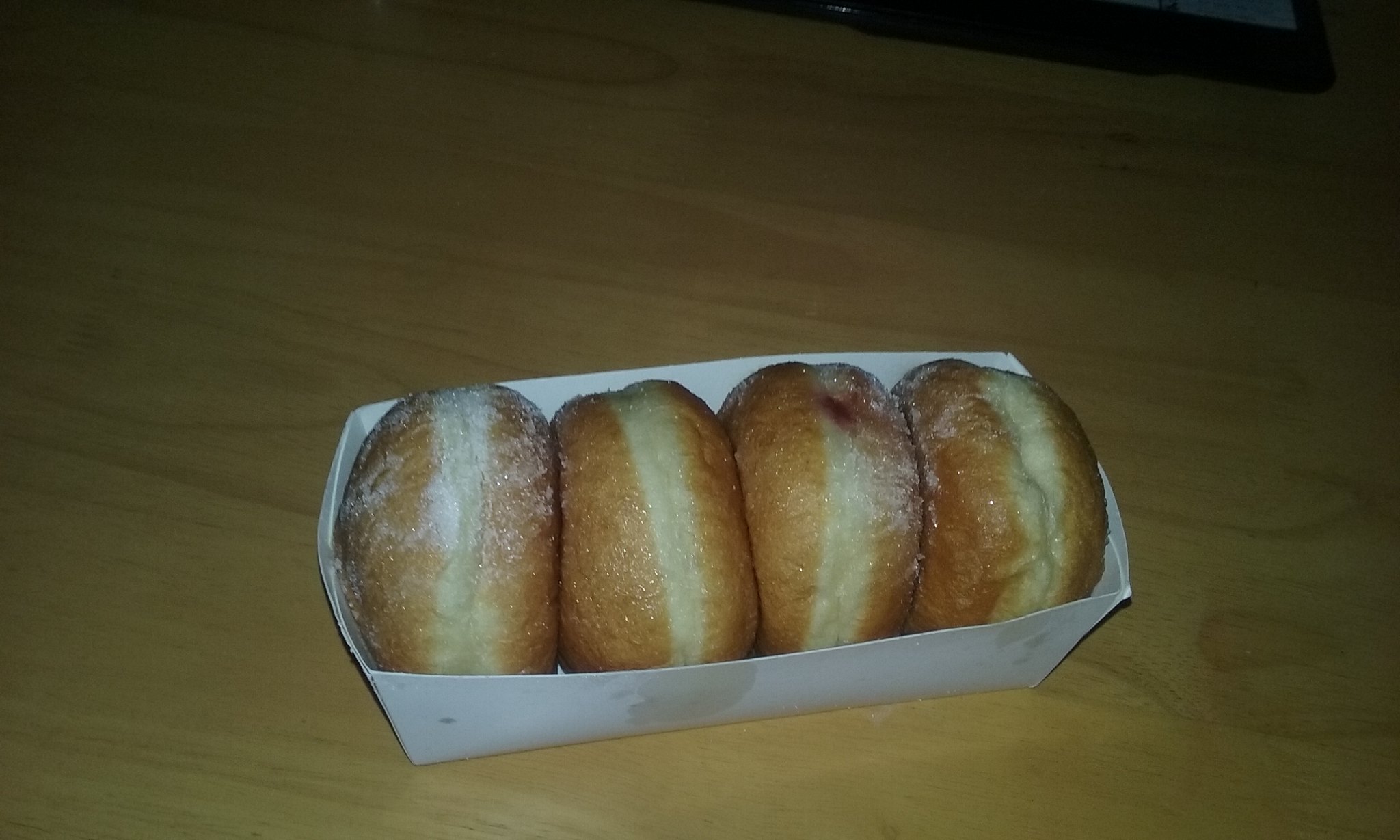This color photograph captures a white paper takeout tray with high sides holding four fresh jelly doughnuts. The photo is shot in a landscape orientation and viewed slightly from above. The background is a light-colored wooden table, possibly made of maple or birch. The table's tan to light brown color contrasts with the darker, shadowed edges of the image. The doughnuts, dusted with fine granulated sugar, are arranged vertically within the tray. Two doughnuts have visible fillings; one has a purplish-red spot indicating raspberry jelly, and the other shows an amber hue, possibly peach filling. The tray itself shows some grease stains. The central subject of the photograph is well-lit, revealing the texture and inviting appearance of the doughnuts, whereas the perimeter remains poorly lit, adding a vignette effect to the image. There is a dark, indistinguishable object near the upper right corner, adding some mystery to the otherwise simplistic and appetizing scene.